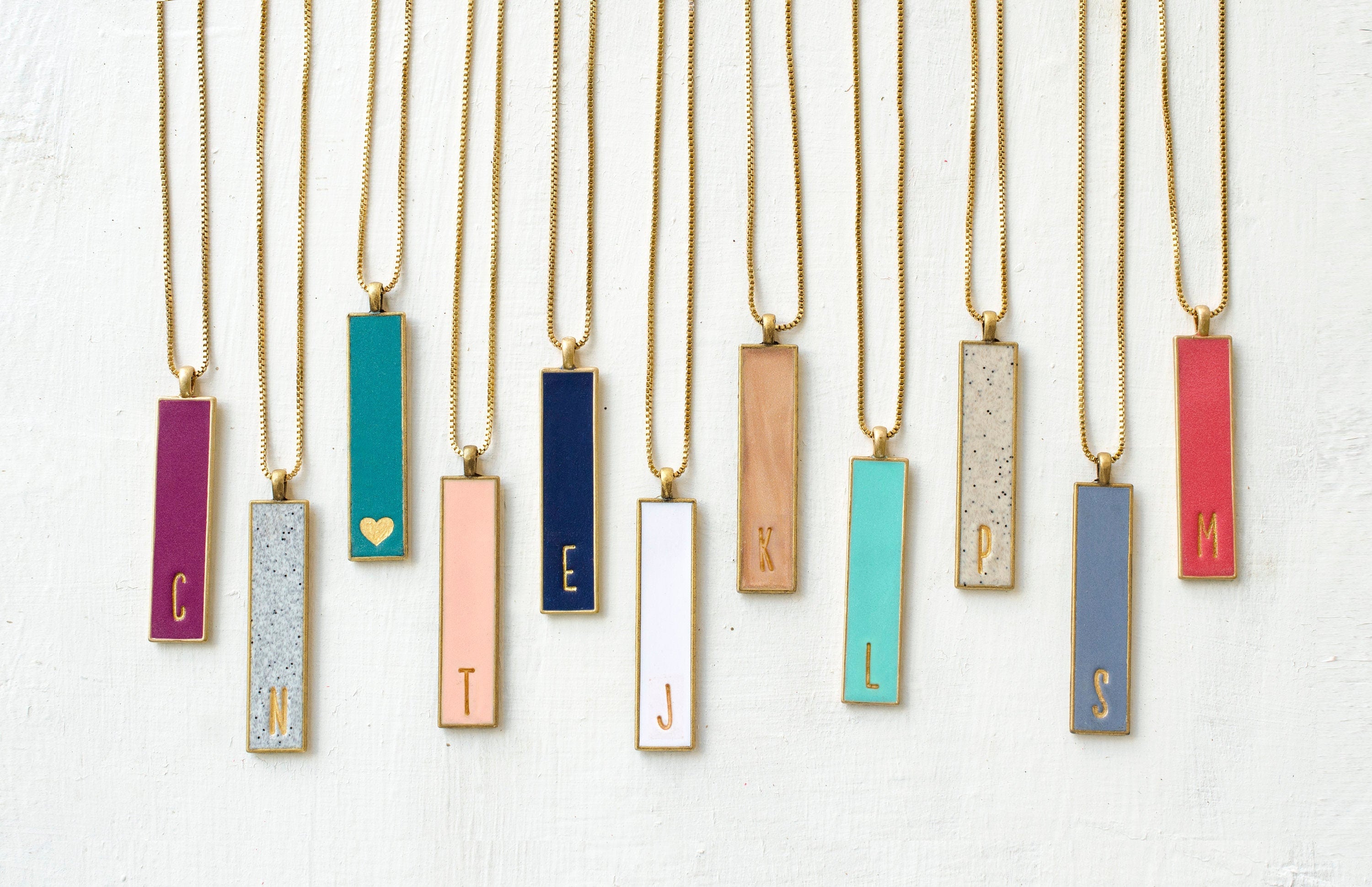The image features a collection of beautifully crafted rectangular pendants, each measuring approximately two inches in length and set on elegant gold chains. The pendants, which hang at varying heights on a white stand, are adorned with either single initials or a small gold heart at the bottom. The pendants showcase a variety of colors and patterns, and each is enclosed in a gold outline with gold hardware attaching them to the chain. From left to right, we see pendants with the following details: a darker purple pendant with a gold letter C, a blue and white speckled pendant with a gold letter N, a turquoise blue pendant with a gold heart, a pink pendant with a gold letter T, a dark blue pendant with a gold letter E, a white pendant with a gold letter J, a peach-colored pendant with a gold letter K, a light blue pendant with a gold letter L, a pink and blue speckled pendant with a gold letter P, a powder blue pendant with a gold letter S, and a pink pendant with a gold letter M. The intricate design and variety of colors make this collection truly eye-catching.